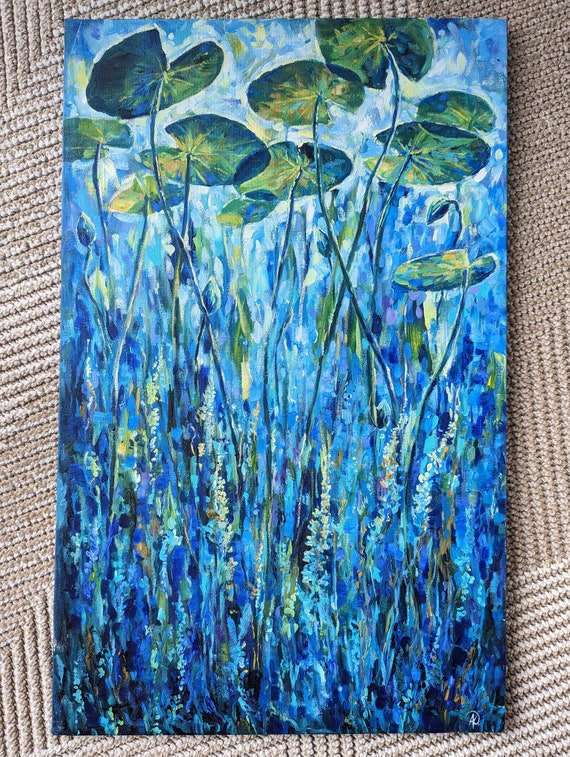This image depicts a rectangular painting resting on a tightly woven, tan-colored jute rug with braided textures and gray lines running at the bottom. The painting features a vivid blue background with various shades of blue, ranging from lighter azure tones near the top to deeper blue hues at the bottom, mimicking an underwater scene. At the top of the canvas, green lily pads float as though on the surface of a lake, their long, slender stems trailing down through the water. This gives the impression of looking up from beneath the water, with the sunlight filtering down. The stems intertwine with what appears to be bluebonnets or sea kelp, enhancing the aquatic theme. Midway up the canvas, there are narrow white flowers or unopened buds, adding delicate details to the vegetation. The green accents and brush strokes scattered throughout the painting contribute to the overall sense of an underwater ecosystem filled with life. The entire artwork, though unsigned, sits compellingly atop the textured jute rug, creating a striking contrast between the natural fibers and the vivid, aquatic imagery.